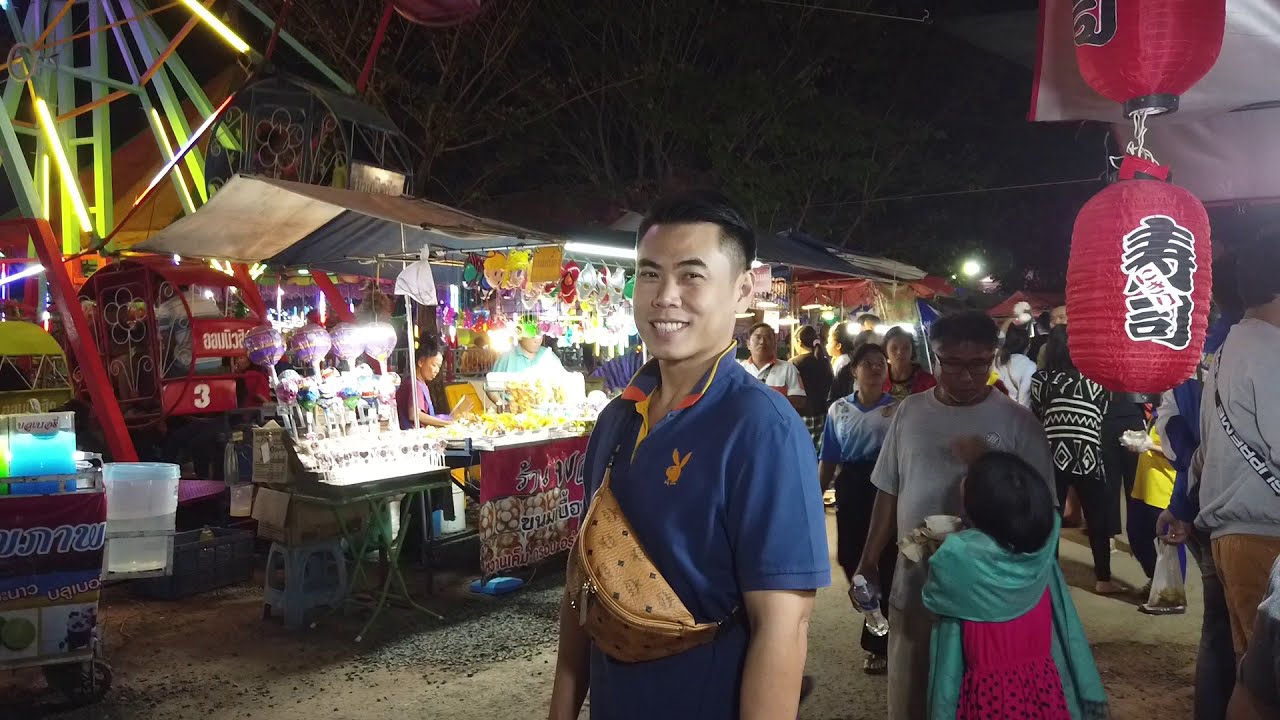A vibrant, full-color photograph captures the lively atmosphere of an Asian night market or carnival, illuminated against a dark, starlit sky. The scene is bustling with activity, highlighted by vibrant red paper lanterns adorned with black Chinese characters and numerous brightly lit stalls displaying souvenirs and food items. On the far left, the illuminated girders and cars of a Ferris wheel add to the festive setting.

Centrally framed in the foreground stands a young Asian male with short black hair, the sides of his head neatly shaved just above the ears. He wears a blue polo shirt featuring a distinctive yellow Playboy Bunny logo on the chest, complemented by a yellow button placket and red and yellow accents on the collar. Draped across his chest is a tan leather man-purse, strapped diagonally like a crossbody bag. His poised demeanor suggests he is aware of the camera. 

Behind him, a little girl gazes up at an older man, possibly inquiring about candy or money, while a cluster of people move through the thoroughfare. An ice cone machine is also visible among the many stands that appear to be selling a variety of treats. The overall scene vividly conveys the dynamic, engaging atmosphere of an Asian festival at night.